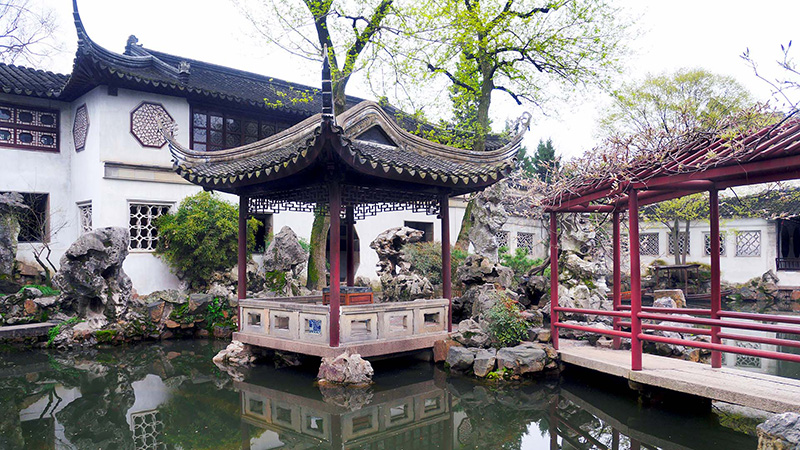This detailed photograph showcases an Asian-inspired setting featuring intricate architecture and serene natural elements. Central to the scene is a picturesque pond with a rectangular pergola or gazebo-like structure, characterized by a distinct black roof that curves upward at the edges and resting on large stones in the water. Adjacent to this structure is a striking walkway or bridge, framed by red poles and tan pathways, extending towards another similarly styled structure, emphasizing the pond's tranquility with dark blue and brown hues. In the background, a prominent white building with a black, pointed roof reflects traditional Japanese design, further echoing the intricacy and elegance of the scene. A stone wall with intricately designed windows frames the backdrop, completing the harmonious blend of architecture and nature, all under a light white sky.